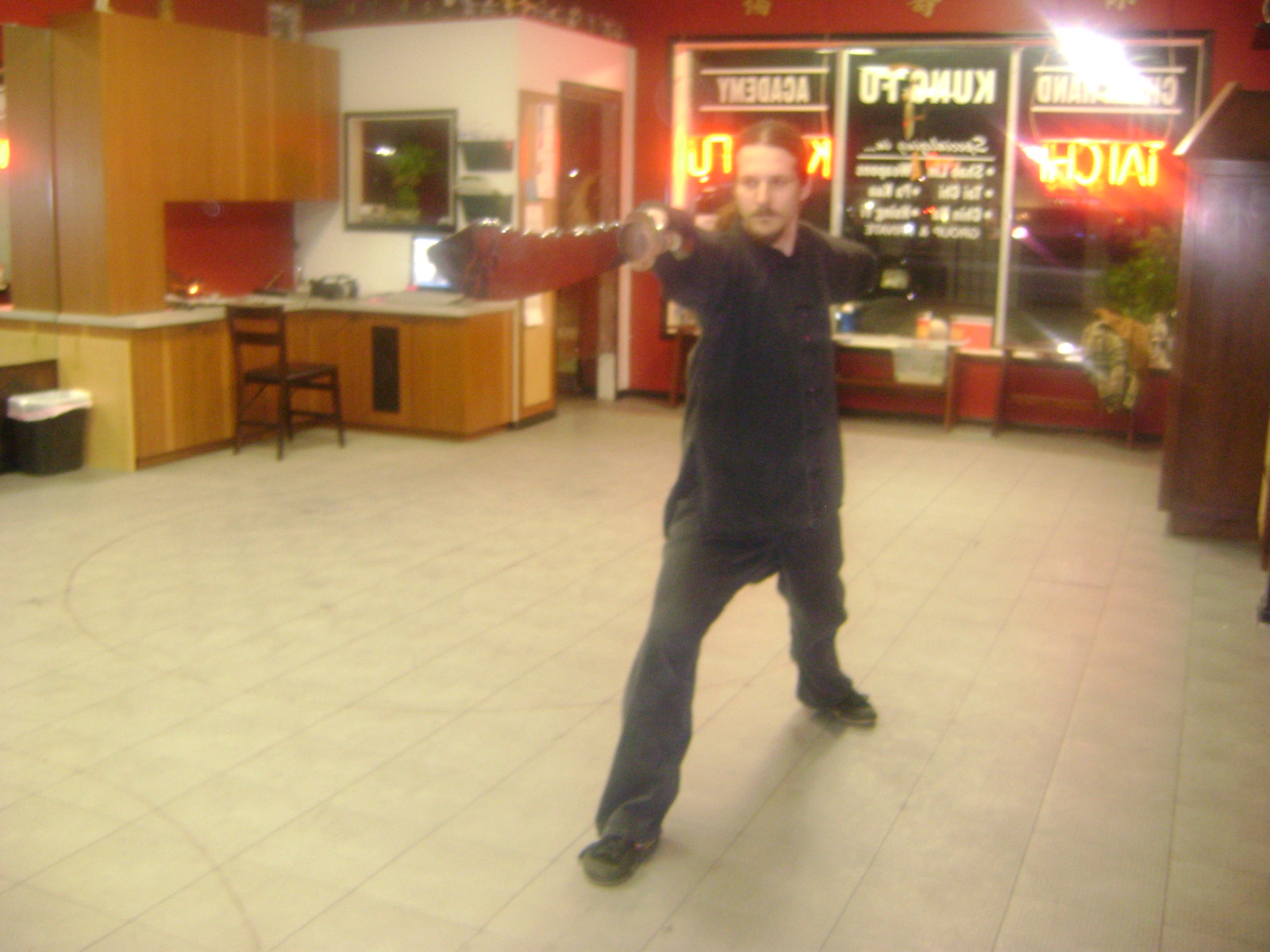This image features a Caucasian man with long brown hair pulled back into a ponytail, standing in a spacious room that resembles a martial arts training academy or potentially a Chinese restaurant, given the décor and ambiance. He is dressed in an Asian-inspired outfit with black pants, a dark shirt, black sneakers, and a distinctive robe-like top that buttons down the middle. The man is striking a pose with his legs spread apart and one arm extended forward, holding a long, metallic silver sword, while his other arm is positioned behind him. The room has a light-colored tile floor and contains a black chair, a counter, a trash can, and a doorway leading to another area. There are windows at the front with white decals displaying words like "Kung Fu" and "Academy," though they are read in reverse from the inside. Neon lights are visible through the windows, adding a bright, vibrant touch to the overall setting.